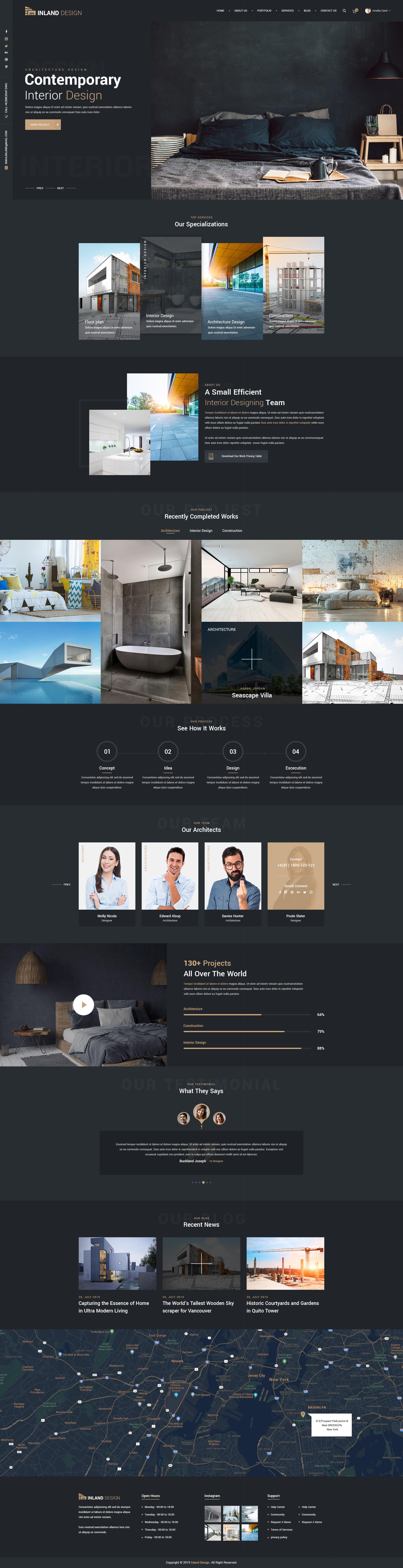**Caption:** 

"This vertical image features a background composed of alternating horizontal blocks in black and dark gray, resembling a tightly compressed snip of a website. At the top, the white text 'Contemporary' stands out against the dark background. Below this header, an image of a bed with gray sheets and pillows is prominently displayed. Beneath the bed image, there are four smaller pictures followed by two additional images, though their contents are indistinct, one of which seems to depict a pool. Just below the midpoint of the page, three individuals are prominently featured, likely indicating they are the designers, realtors, or builders associated with the website. The overall layout and content suggest this is a webpage for a developer, home builder, or designer."